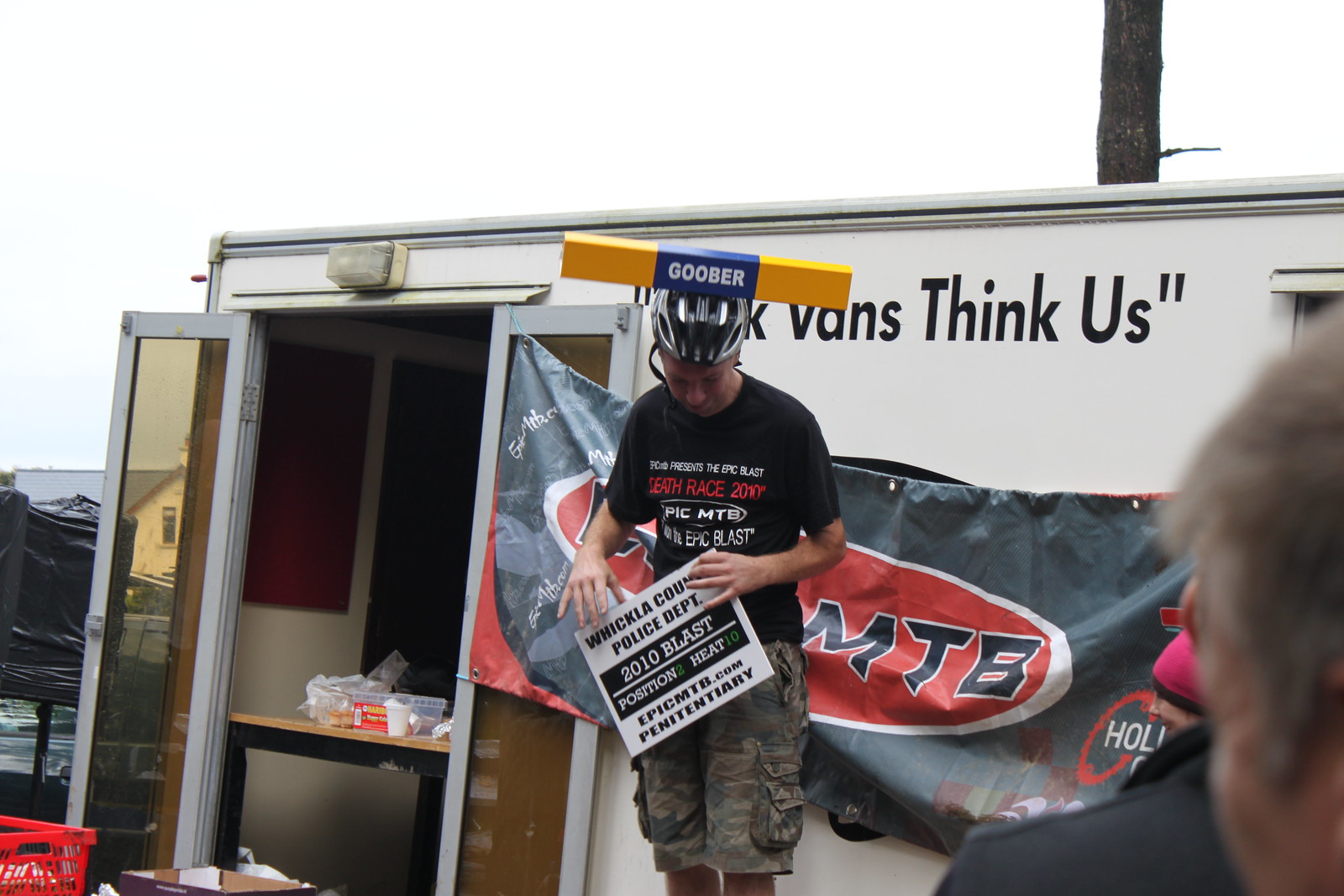The photograph captures a man standing at the center, wearing a distinctive black helmet with a yellow block on top. This block has dark blue in the middle and the word "Goober" in white text. The man is looking down and dressed in a black t-shirt, partly obscured by a sign that reads "Wicola County Police Department 2010 blast Position Something heat 10," along with other indecipherable text. His t-shirt also has unreadable text in a mix of white and red. He is wearing camouflaged cargo shorts, with his lower legs cropped out of the image.  

Behind him is an open trailer with double doors to the left. One of the doors has a black banner with a red oval logo, partially obscured by the man. Some text on the trailer reads "VANS THINK US" in parentheses, though the rest is also obscured. To the right, there is a slightly blurry, close-up image of another man's face with grayish hair, along with the face of a woman in the background, wearing a pink beanie. The sky above is overcast with an off-white hue.

There is a table with black legs and a light brown surface to the left of the trailer, possibly holding some snacks. Additionally, there is a red basket at the bottom left corner of the image and a few trees are visible behind the trailer. The setting appears to be outdoors during a cloudy day.